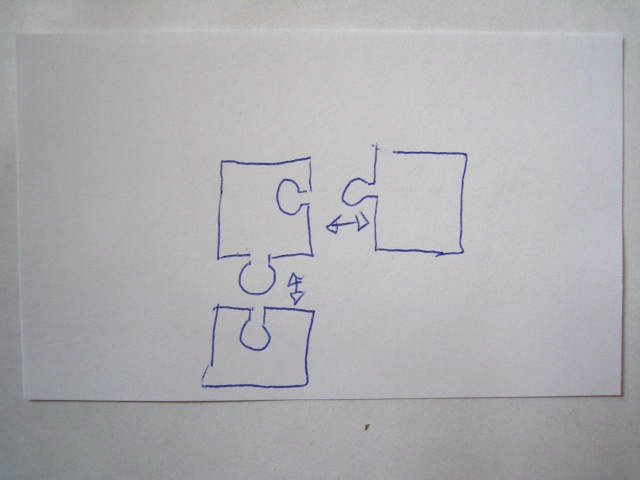A detailed drawing on an elongated piece of white paper, approximately 8.5 by 13 inches, rendered in blue ink. The illustration depicts the outlines of three jigsaw puzzle pieces, arranged in a linear fashion. The central piece connects seamlessly to the pieces on either side, resembling a small segment of a four-piece jigsaw puzzle.

The top puzzle piece features an extended tab that fits into an adjacent empty space of the middle piece. Between the top and middle pieces, a double-sided arrow indicates their compatibility and alignment. Similarly, the center piece extends a tab into a corresponding space in the bottom piece, with another double-sided arrow illustrating their interlocking nature.

Each jigsaw piece is characterized by a plain outline, with tabs and spaces designed for interconnection. However, the bottom and side edges of these pieces are flat, implying a lack of further connectivity beyond this three-piece assembly. The arrows accentuate the idea that these pieces can fit together, yet the design suggests limitations in forming a comprehensive puzzle.